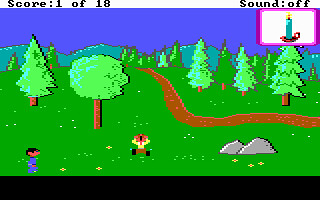This image is a color screenshot from an NES-era 2D platformer video game, characterized by pixelated and dated graphics typical of the 80s or 90s. At the top left, it prominently displays a score of 1 out of 18, and in the top right, it indicates that the sound is off. There's a pink box in the upper right-hand corner containing a lit green candle on a candle holder with a looped handhold. The scene features a detailed forest landscape, including a variety of roundish leaf trees, pine trees, and a mountain range with visible mountain lines. A dark brown path cuts through the grass, adorned with flowers and scattered gray rocks. In the bottom left corner, a figure in a blue jumpsuit with black hair is seen walking, while another figure in brown pants and a yellow shirt is lying on the grass with arms extended as if screaming. The graphics are notably primitive, reminiscent of early computer games.